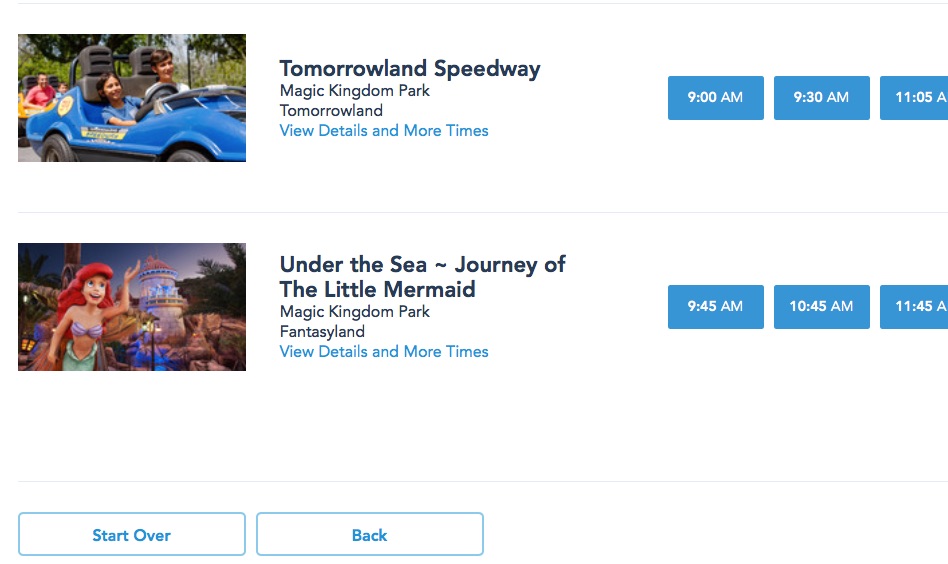In the detailed image, on the right side, there is a vibrant photograph featuring a boy and a girl seated in a blue go-kart. Behind them, another picture showcases a man with a young child in a yellow go-kart. Above this scene, in bold black lettering, the sign reads "Tomorrowland Speedway," indicating its location in Magic Kingdom Park's Tomorrowland. Adjacent to this, a section displays more information and times in blue text, with three blue boxes below listing available times: 9:00 a.m., 9:30 a.m., and 11:05 a.m.

Below this, another engaging image captures the Little Mermaid, recognizable by her red hair, purple shell top, and green tail fin. She is depicted with her left hand raised and her right arm lowered. The background includes an enchanting combination of trees, rocks, light poles, and a scenic area featuring rocks and a winding bridge. In black lettering, the text reads "Under the Sea, Journey of the Little Mermaid, Magic Kingdom Park, Fantasyland." Additional details and timings are provided in blue text next to three available time slots: 9:45 a.m., 10:45 a.m., and 11:45 a.m.

At the bottom of the image, there are two semi-long rectangular buttons outlined in blue with white backgrounds and blue lettering. One button reads "Start Over," and the other says "Back."